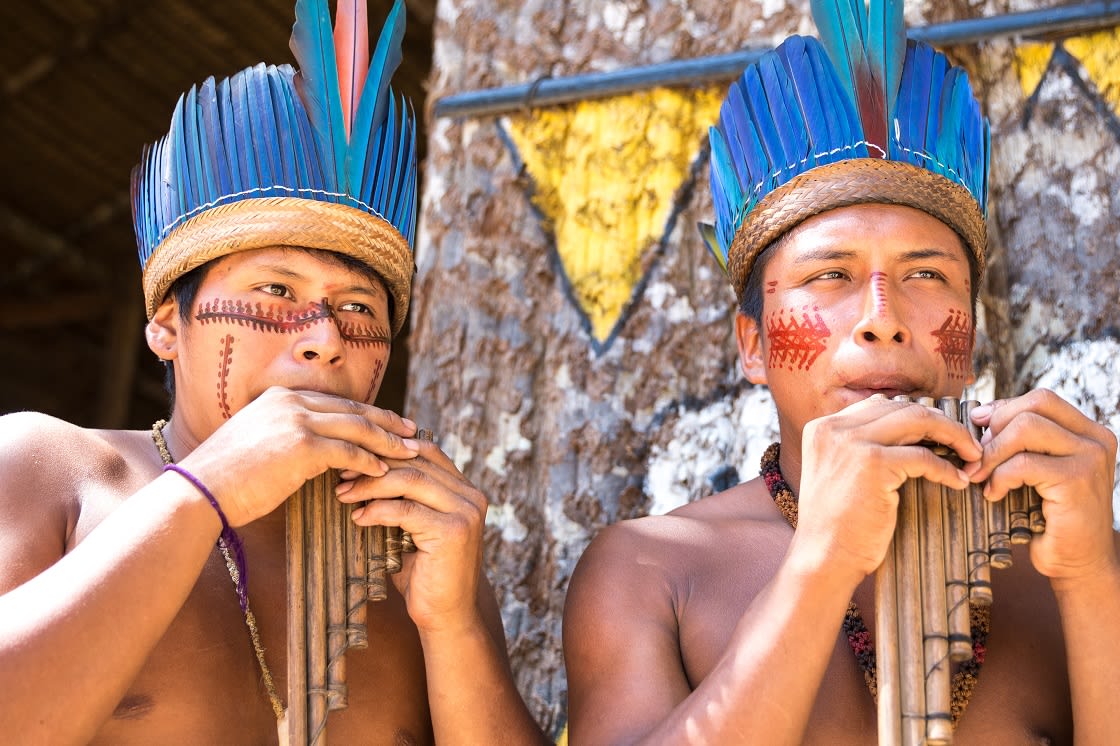The image depicts two young men, likely of indigenous descent, playing hand-carved pan flutes. Both are shown from the chest up and are bare-chested. They adorn intricate headdresses made of blue feathers, possibly from birds of paradise, with a woven tan band at the base. They each wear face paint: the man on the right has red paint with several short lines on his nose and cheeks, and the man on the left features a black and red design stretching horizontally beneath his eyes, in addition to vertical lines on his cheeks. The man on the right is adorned with a colorful necklace of yellow, pink, and green hues, while the man on the left sports a simpler, twisted twine necklace and a purple bracelet. The backdrop includes a rough-barked tree or possibly a wooden wall, decorated with yellow inverted triangles and lichen, enhancing the rustic and cultural ambiance of the scene. Both men have dark eyes and medium complexions, encapsulating a striking and evocative image of traditional indigenous culture.